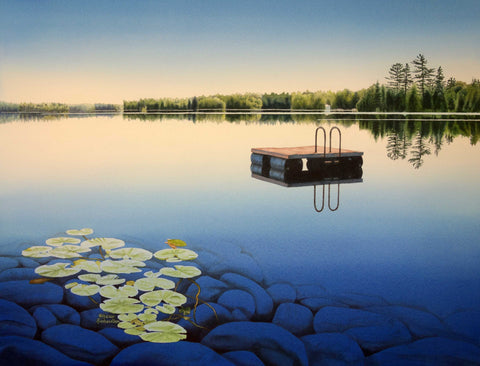The image captures a tranquil lake scene under a gradient sky transitioning from a golden peach hue at the horizon to a rich dark blue overhead. In the center of the lake, a wooden barge-like platform floats, equipped with a ladder. The bottom left corner of the image showcases green, circular lily pads with bluish stones beneath them, reflecting the water’s color. Surrounding the lake, the shoreline is dense with green trees, including a mix of evergreens and broader-leaved varieties. In the far distance to the right, taller trees stand out, completing this serene natural setting.